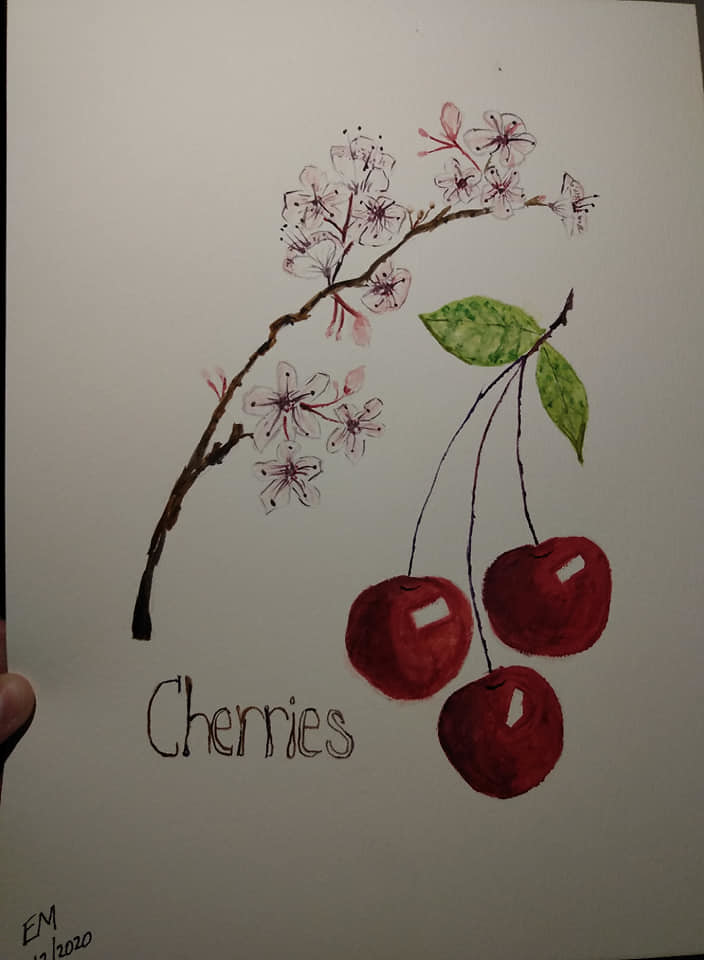This detailed image features a meticulously crafted painting on a white piece of paper, held at the bottom left by the visible tip of a thumb. The artwork showcases two distinct elements: a branch of cherry blossoms and a cluster of cherries. The cherry blossom branch starts slightly toward the bottom left and gracefully arcs upward to the top right, adorned with approximately 10 to 12 blooms in shades of soft pink and bolder pink highlights. On the right side, three vibrant red cherries dangle from individual stems that converge at a small branch, accompanied by two rich green leaves. Each cherry is marked with a small white rectangle to depict its shine. Below the cherries, the word “CHERRIES” is inscribed in capital and lower-case letters as "Cherries." In the lower left corner, the artist's signature, "EM," is visible, although the date beneath it is partially obscured but indicates the year 2020. This composition cohesively integrates the delicate beauty of cherry blossoms with the bold, ripe appeal of cherries, blending them into a harmonious visual narrative.